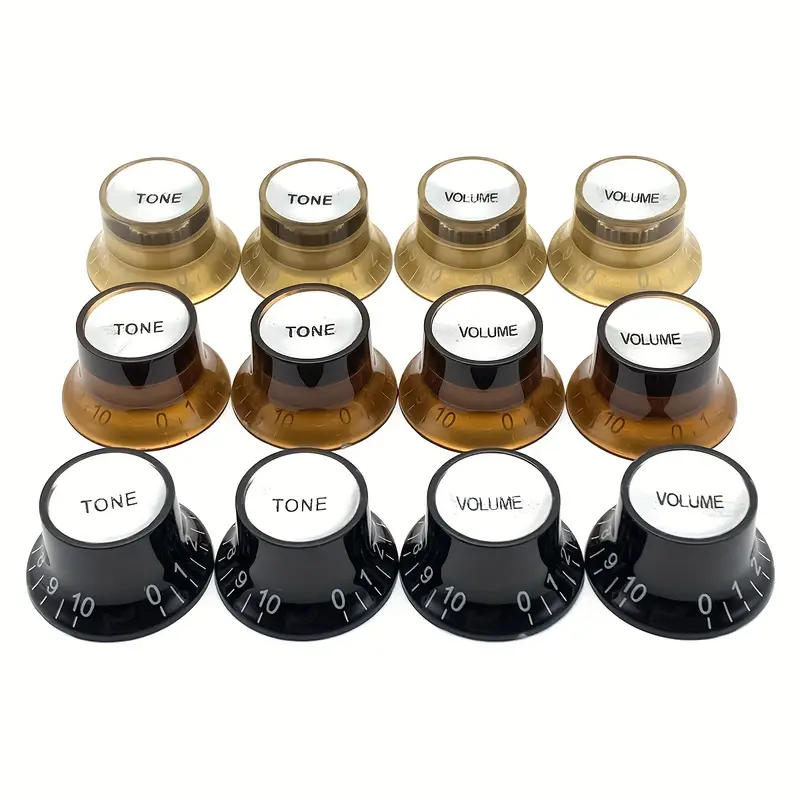The image showcases an arrangement of 12 control knobs arranged in three rows of four. Each row features two "TONE" knobs on the left and two "VOLUME" knobs on the right. The top row contains brass-colored knobs with black lettering for the labels and raised gold numbers around the edges. The middle row consists of darker, bronze-colored knobs that similarly display "TONE" and "VOLUME" labels, with brown numbers around the edges. The bottom row features black knobs with white numbering encircling the edges, maintaining the consistent labeling format of "TONE" on the left and "VOLUME" on the right. The knobs are organized on a white background, possibly intended for a product feature display.